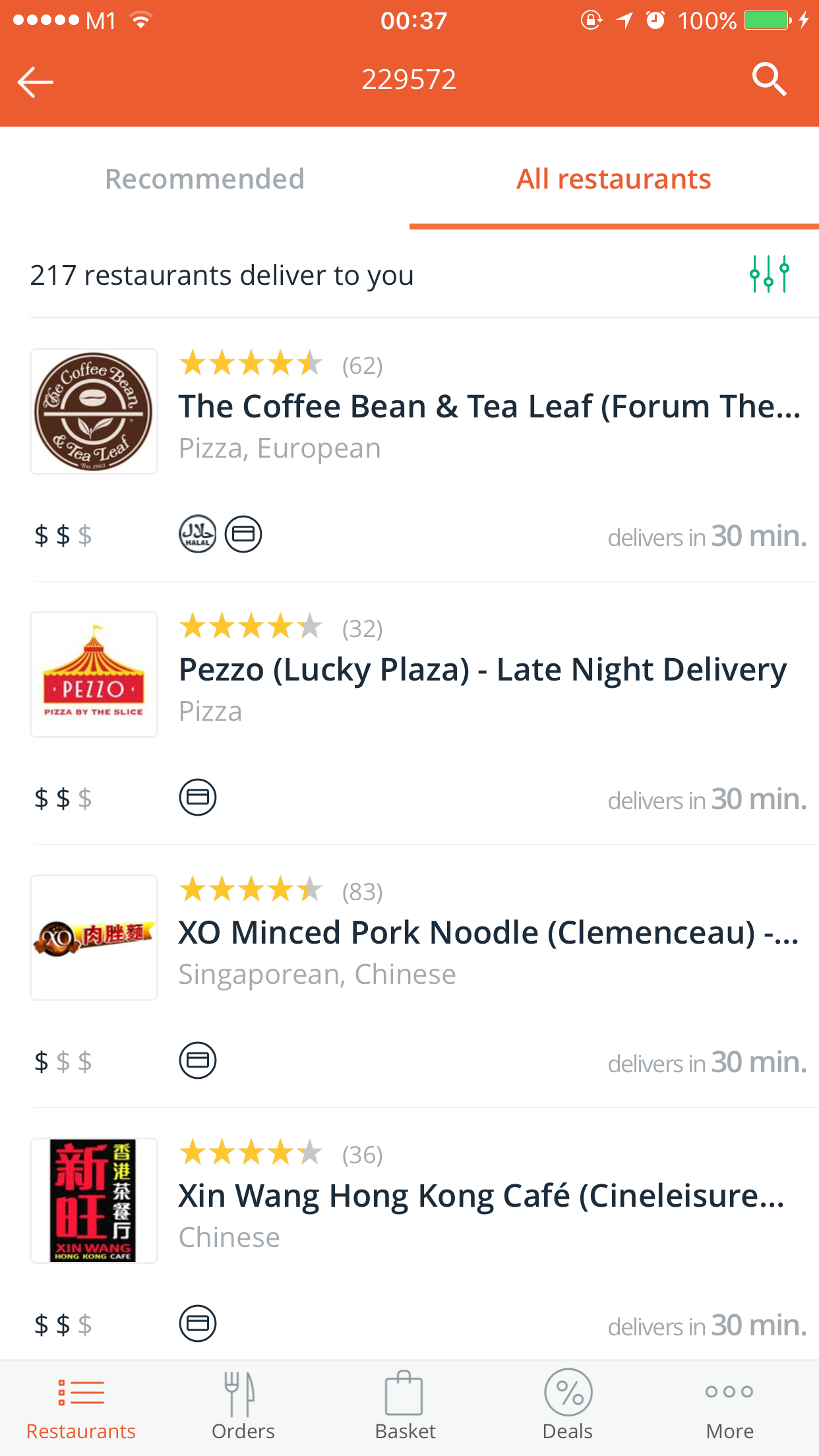The image depicts the interface of a food delivery app on a smartphone screen. At the top left corner, there are several white dots followed by the text "M1" and a Wi-Fi signal icon. Centrally, the timer displays "00:37", while the top right corner features a lock icon enclosed in a circle, a white arrow, an alarm clock icon, "100%" battery percentage, and a green battery icon.

Below this, in a prominent orange section with white text, the number "229572" is displayed. To the left of this number is a left-pointing white arrow and to the right, a white magnifying glass icon.

Further down, two tabs are situated— "Recommended" in gray and "All Restaurants" in orange, with an orange underline indicating the selected tab. Underneath, a line of text reads "217 restaurants delivered to you."

The list of restaurants begins with "The Coffee Bean & Tea Leaf", followed by the word "(Forum)" partially cut off. Its cuisine is labeled as "Pizza, European", and it features a brown icon to the left. The delivery time is stated as "Deliver in 30 minutes" with a price range indicated by two out of three dollar signs.

Next is "Pe$o Lucky Plaza" under the "Late Night Delivery" section. It has garnered four stars from 30 or 32 reviews.

Following that is "Exo Minced Pork Noodle Clemenceau," categorized under "Singaporean, Chinese."

Lastly, "Xin Wong Hong Kong Cafe" at "Sina Leisure" offers Chinese cuisine. 

At the bottom of the screen, navigation icons labeled as "Restaurants," "Orders," "Basket," "Deals," and "More" are visible.